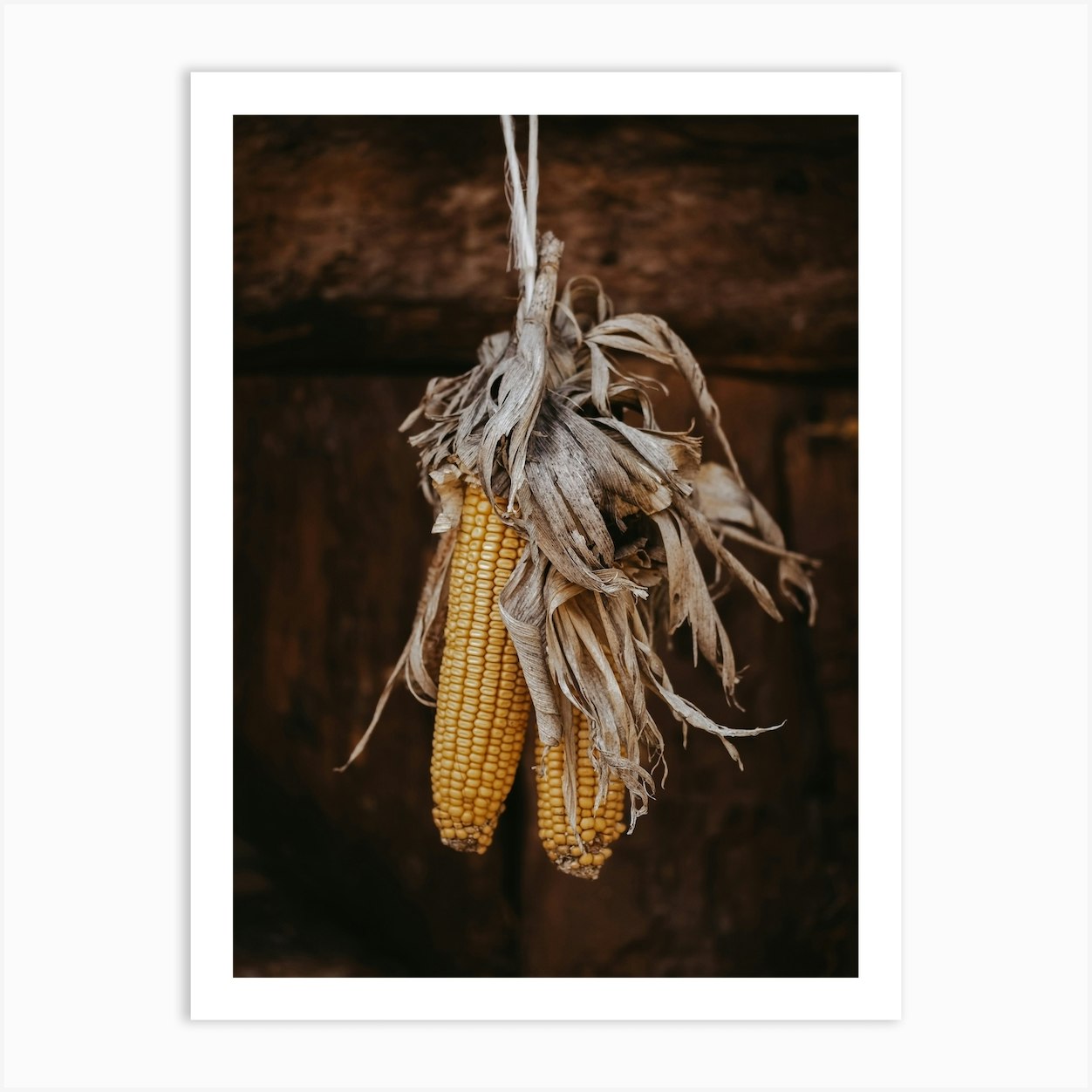This detailed photograph features a vertically rectangular image encased within a broader square frame that is slightly off-white, creating a distinct visual contrast. The image itself is bordered by a thicker light gray margin followed by a thinner white border. Within these borders lies a dark, mottled brown backdrop, resembling an aged wooden door. Central to the photograph, two ears of dried yellow corn hang upside down from a discreetly positioned hook via a piece of rope. The kernels, hardened and inedible, evoke the look of traditional Indian corn. Surrounding the corn, the dry, straw-like husks have turned a very light brown or tan color, cascading down and partially obscuring the lower portion of the right ear. This rustic arrangement serves as a fall decoration, exuding a warm, seasonal charm.